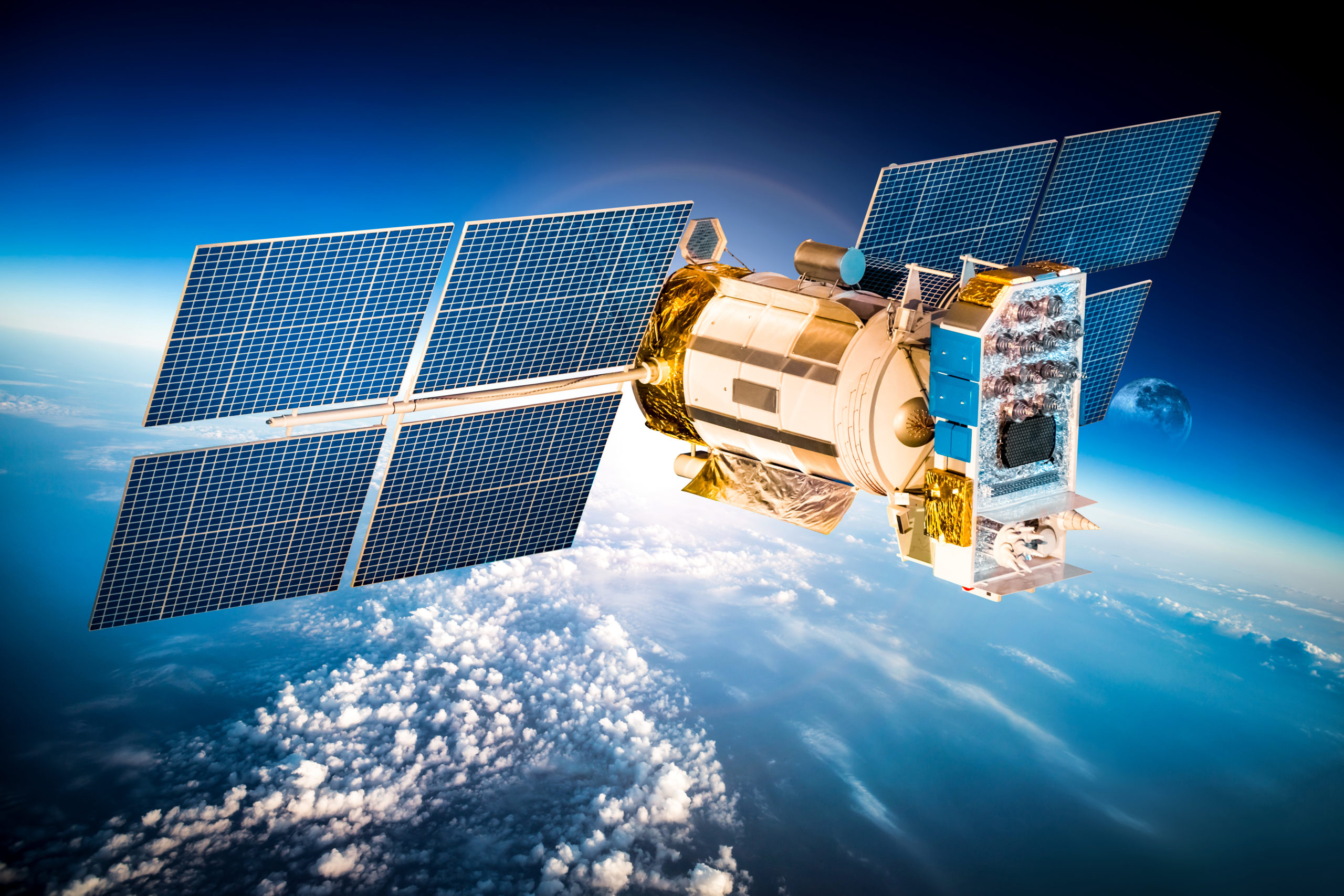A highly detailed digital rendering depicts a satellite orbiting above Earth against the vast expanse of a dark, black sky. The satellite features a prominent white cylinder at its center, with gold sections at both its front and rear. The right side of the satellite is characterized by a rectangular module adorned with white plates on its sides, gold plates on its top, and an electrical board with silver circles at the back. Extending from the main module, large solar panels on either side are held together by a white rod. The left-side solar panels, four in number, boast a dark blue hue with a grid pattern of white lines.

Beneath the satellite, soft white clouds stretch across a vividly blue Earth. To the right, partly obstructed by the satellite’s structure, the Moon appears with a faint blue tint and dark spots. Above and around, rays from the Sun subtly illuminate the scene, casting a gentle glow over the mostly blue and white composition, contrasted by the tan and gold of the satellite's main body and modules. The overall atmosphere of the image — be it a photograph or a digital creation — is serene, highlighting the sophisticated beauty of space exploration technology against the backdrop of our home planet.